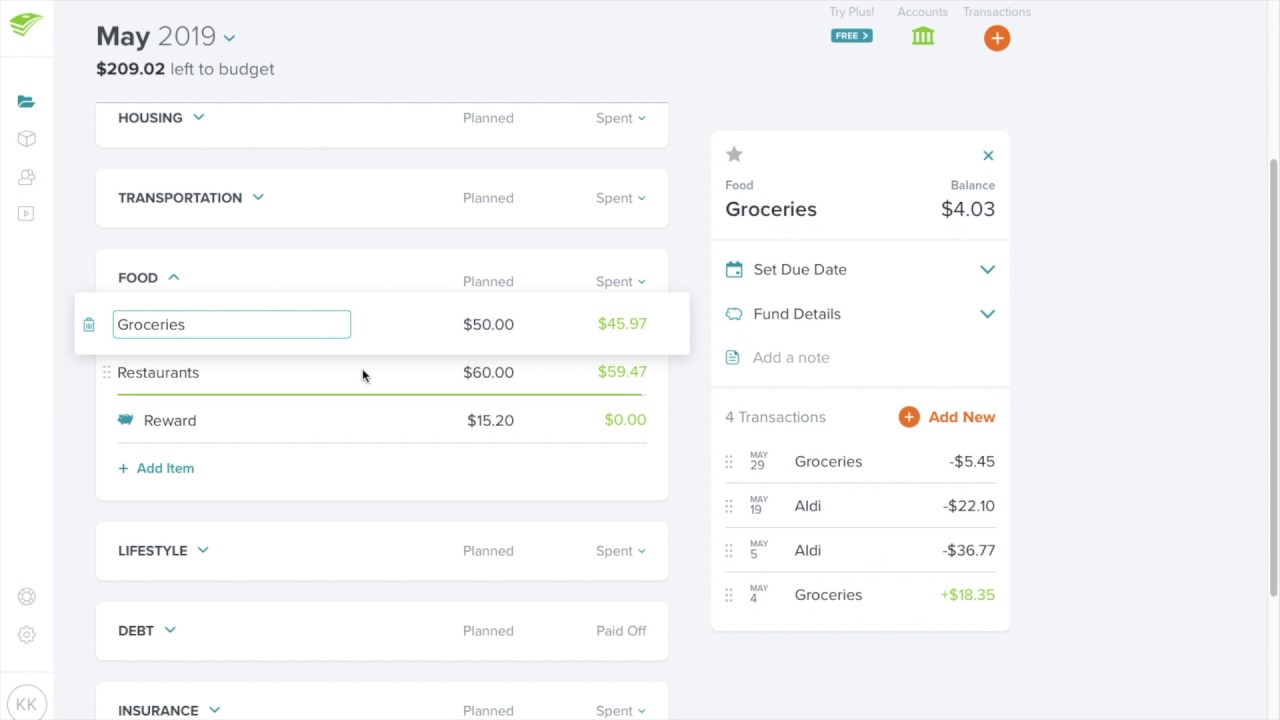This screenshot captures a detailed look at an individual's budget management page, possibly from an application similar to QuickBooks, though not explicitly identified. 

At the top left, there is a distinctive logo featuring a green stack of money. Surrounding this logo are multiple navigation options, including settings, profiles, and other functional categories. Directly across the top, the period of the budget is displayed as May 2019. It is noted that there is $209.02 remaining in the budget for this period.

On the far right, there are prompts to try some software for free, alongside options to manage accounts and list transactions. The central area of the page is devoted to the budget breakdown, categorized into various sections such as Housing, Transportation, Food, Lifestyle, Debt, and Insurance, each with 'Planned' and 'Spent' columns. Both Housing and Transportation have no entries in either column.

Under the Food category, subcategories show detailed budget information. For Groceries, $50 was planned, and $45.97 was spent, leaving a balance of $4.03. For Restaurants, $60 was budgeted, with $59.47 spent. There’s also a Rewards section noted at $15.20, although details are sparse, and an 'Add Item' button is present.

The Lifestyle, Debt, and Insurance categories have no entries for planned or spent amounts. On the far right of the screen, a pop-up related to the Groceries subcategory details that $4.03 is left from the original $50 allocation. The pop-up includes additional features like setting a due date, fund details, and adding new items.

Beneath this, transaction details show four entries, indicating this individual has made multiple purchases at ALDI, tracking their expenditures closely within the groceries budget.